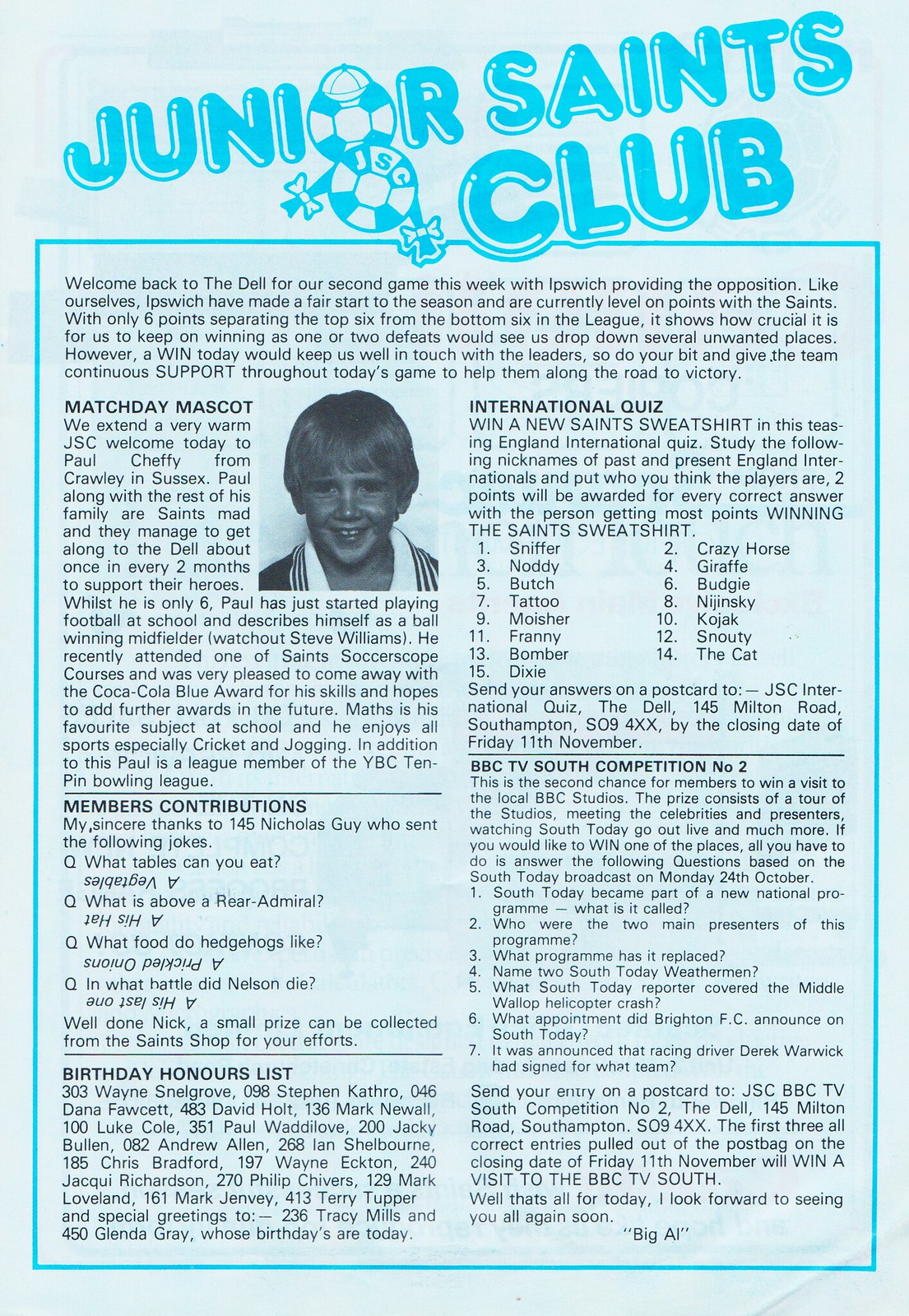The image features a busy newsletter dedicated to the Junior Saints Club, prominently headlined in capital blue letters at the top. Set against a light blue backdrop, the newsletter's content is packed with five distinct articles, extensive paragraphs of text, and various headings that cater to its young audience. 

The foremost article enthusiastically welcomes readers back to the Dell for a second game of the week against Ipswich, elaborating on the importance of wins to maintain their standing in the league. A central feature of the newsletter is a black-and-white photograph of a smiling boy, Paul Chaffee from Crawley in Sussex, who is honored as the Match Day mascot. Additional sections include a heartfelt thanks to member Nicholas Guy for his joke contributions, a list of birthdays, and an international quiz offering a chance to win a new Saints sweatshirt.

Another notable segment announces the BBC TV South competition number two, providing all the details for member participation, including a visit to the local BBC studios for the winners. The newsletter is addressed to the enthusiastic Junior Saints Club community, encouraging continuous support for their soccer team while providing various interactive and celebratory elements for their engagement.